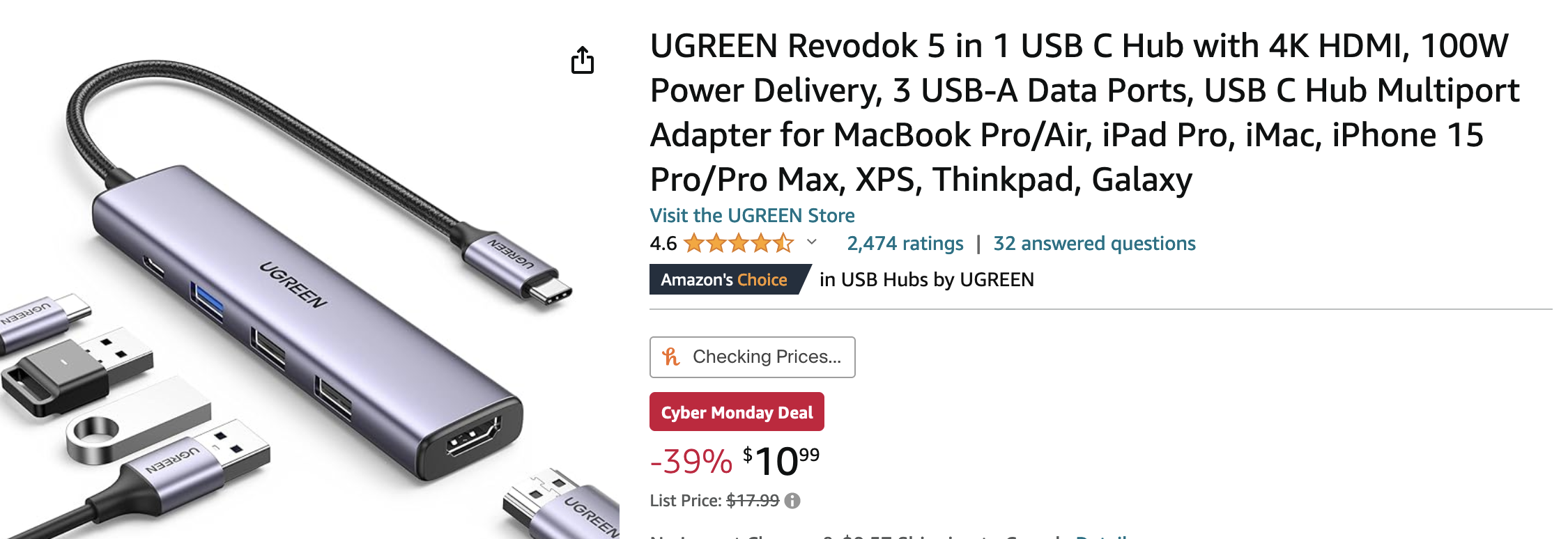The image illustrates a UGREEN RevoDock 5-in-1 USB-C Hub prominently displayed. On the left, a charging cord is visible, featuring a small connector to plug into a power adapter. The cord extends to a sleek, silver rectangular area designed to fit additional connectors. The UGREEN brand name is clearly labeled on both the hub and throughout the description.

The detailed product description to the right highlights the RevoDock's capabilities: 4K HDMI output, 100W power delivery, and 3 USB-A data ports. It serves as a multi-port adapter compatible with various devices, including the MacBook Pro/Air, iPad Pro, iMac, iPhone 15 Pro, XPS, ThinkPad, and Galaxy.

A button labeled "Visit the Ugreen store" is also present. The product boasts a rating of 4.6 out of 5 stars based on 2,474 customer reviews and has 32 answered questions. As an Amazon's Choice item, it features a clickable option to check prices. Additionally, there is a Cyber Monday deal highlighted in red, indicating a 39% discount, bringing the price down to $10.99.